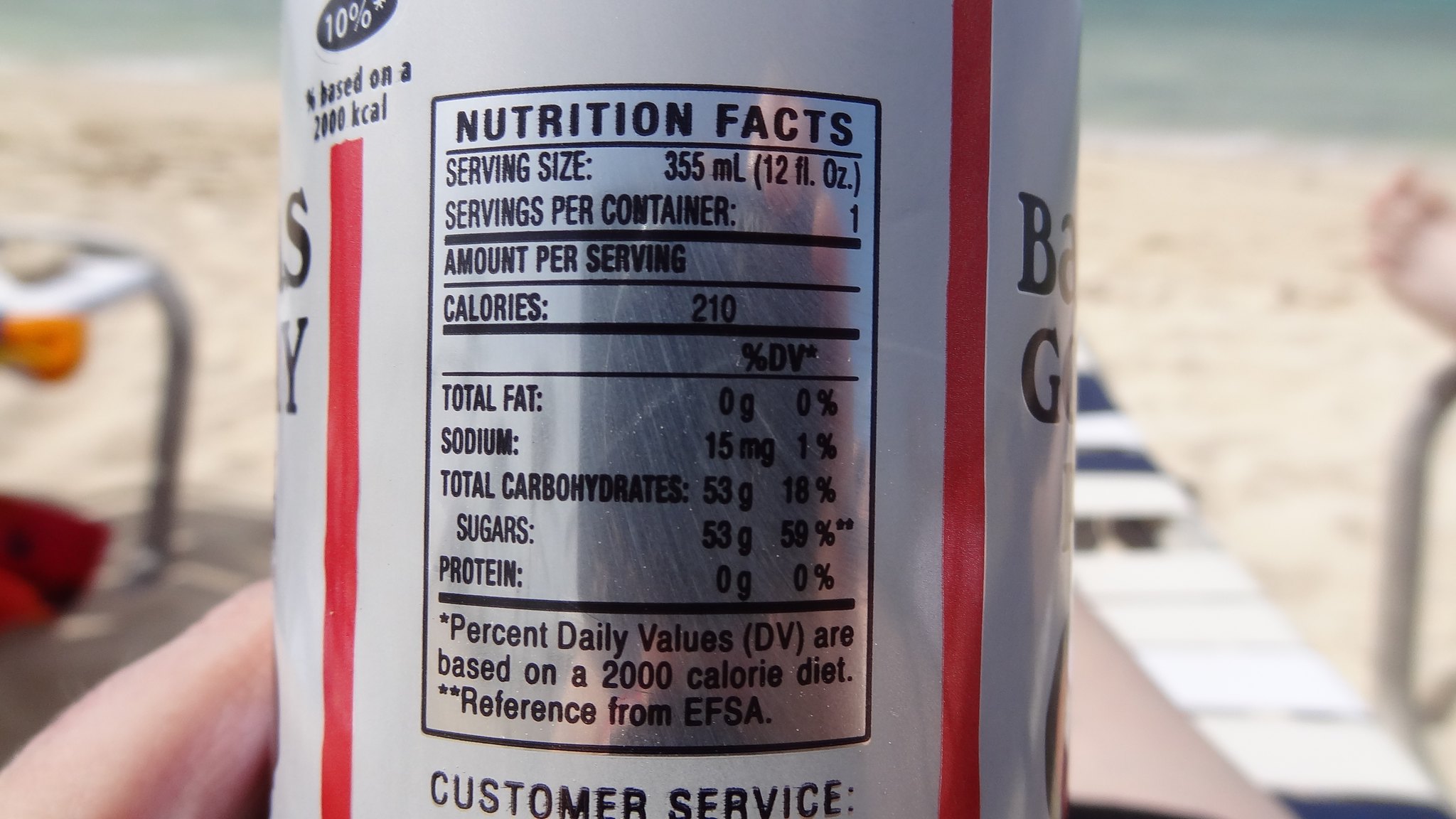A silver beverage can is prominently held up against a scenic beach backdrop. The can features black text and red vertical trims running along its sides. It displays nutritional information in a black-lettered rectangle, listing details such as serving size (355 milliliters), total servings (1), and nutritional content: 210 calories, 0 grams total fat, 15 grams sodium, 53 grams total carbohydrates, 53 grams sugars, and 0 grams protein. In the background, the edge of the beach meets the waterline, with beach chairs and a pair of toes visible on the far right, adding to the relaxed, coastal atmosphere.